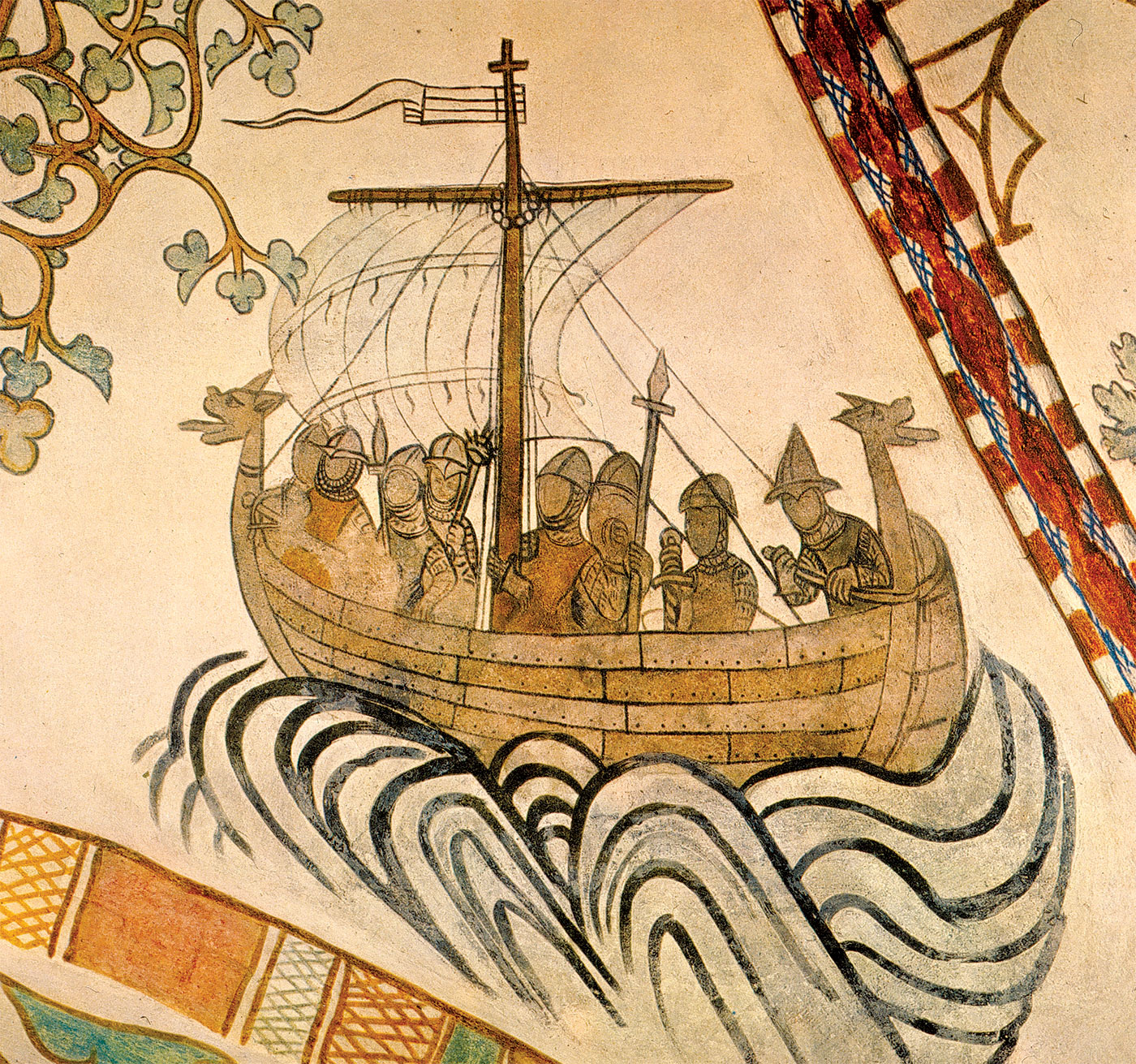The image is a colorful medieval-style painting or drawing, depicting a small, crowded sailboat brimming with various figures. Centrally featured, the boat sports a prominent mast topped with a cross symbol and a white flag. Onboard, a notable figure resembling a pope stands amidst warriors clad in chainmail vests, helmets, and medieval armor, some wielding spears and maces. The soldiers' faces are simplistic, just blank ovals. The vessel itself is adorned with animal figureheads—likely dogs or dragons—facing in opposite directions. The waves underneath are illustrated with black and white curvy lines, adding a dynamic motion effect. The scene is framed with decorative borders featuring a mix of red, white, blue, orange, yellow, and green hues. Completing the composition, a tree branch with leaves extends into the image from the top left corner.